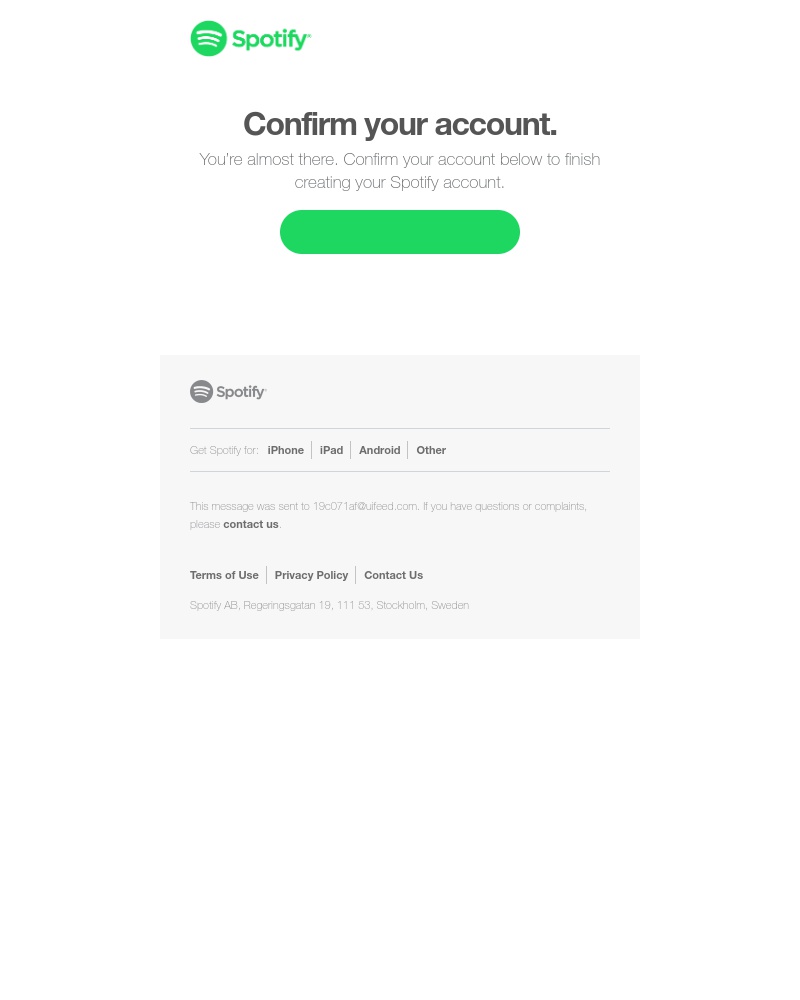Screenshot of Spotify Account Confirmation Email:

The screenshot captures the account confirmation page for Spotify. In the upper left corner, the recognizable Spotify logo is displayed in its green color. Central to the screen is a prominent, bold black text that reads: "Confirm your account." Below this header, a message states, "You're almost there. Confirm your account below to finish creating your Spotify account." Immediately following this instruction is a green call-to-action button; however, it is noteworthy that the button lacks any visible text at the moment.

This image appears to be a screenshot from an email communication. Directly beneath the call-to-action button, there is a gray footer section. The Spotify logo is again present here, but it is displayed in a gray hue rather than green. Within this footer, there are various links provided for the convenience of the recipient: "GetSpotify for iPhone, iPad, Android, or other." Further down, text in a lighter gray font indicates, "This message was sent to [an email address]. If you have questions or complaints, please contact us."

Finally, near the bottom of the message, links to "Terms of Use," "Privacy Policy," and "Contact Us" are listed. The very end of the email contains Spotify’s business address located in Stockholm, Sweden.